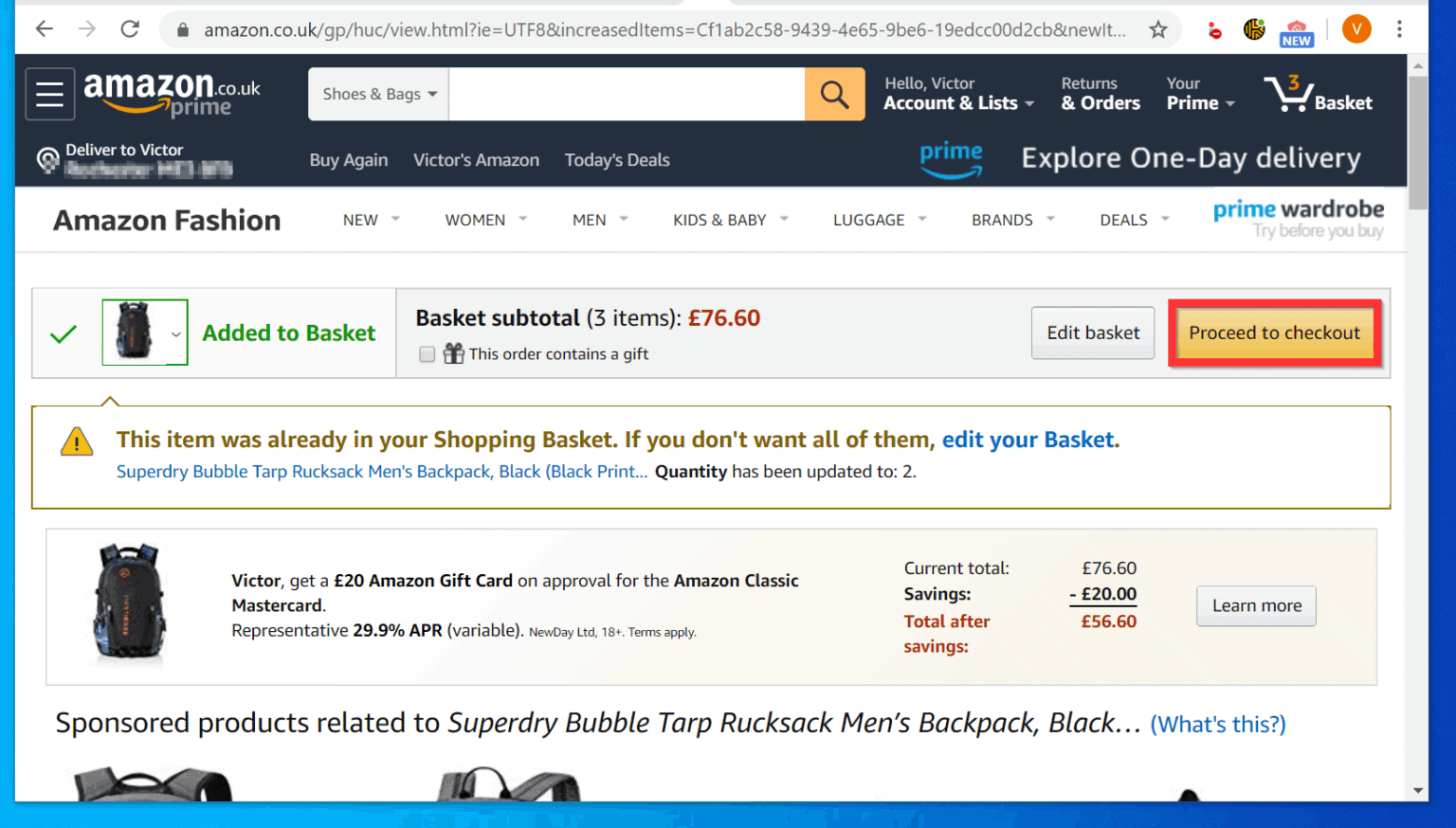This is a minimized screenshot of an amazon.com UK desktop webpage displaying the "Proceed to Checkout" page. At the very top, the taskbar shows "amazon.com UK" in the search bar, containing the website address. The page has a white background and, on the left side, text reads "Item added to basket" accompanied by a green checkmark, confirming the addition. Below this, there is a thumbnail of a backpack. To the right, it states "Basket subtotal (3 items)" with the total price underneath. A checkbox labeled "This order contains a gift" is present but not selected. Further to the right, options read "Edit Basket" and "Proceed to Checkout," the latter highlighted with a red rectangle indicating it as the next action step. Below this section, a banner alerts, "This item was already in your shopping basket. If you don't want all of them, edit your basket." Towards the bottom, there is a larger thumbnail of the same backpack with a promotional message to its right stating, "Get a $20 Amazon gift card if you're approved for the Amazon MasterCard."